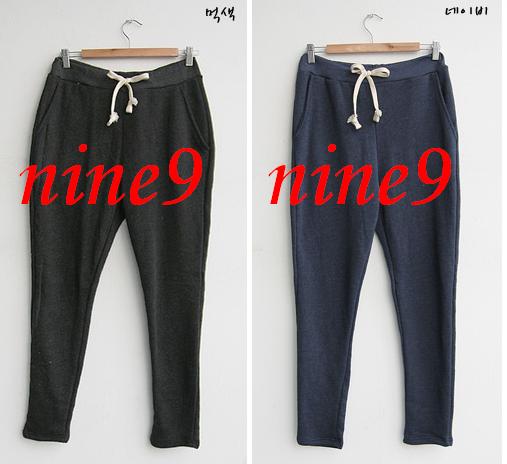In this square-format, color photograph, there are two side-by-side images of trousers, resembling pajama or jogger pants. Both pairs of trousers hang from wooden and metal clothes hangers with clips. The trousers are displayed against a neutral background. They feature a slim fit and are designed to taper at the ankles. Each pair has a white drawstring for adjusting the elastic waistband. The left pair is black, while the right pair is a grayish blue. Overlapping the front of each image is bold red text reading "NINE 9." The pants appear soft and informal, potentially suitable for casual or lounge wear. Additionally, there are black squiggles in the top right corner of each photo, adding a decorative element to the advertisement.